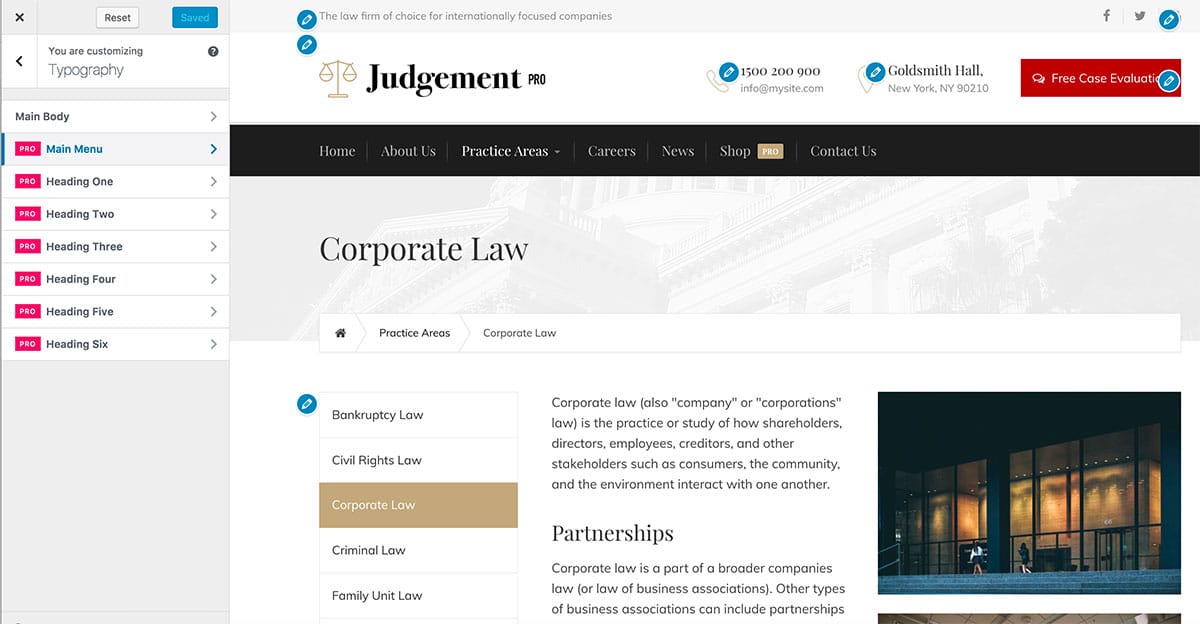In the image, the top section displays the text "Reset" and "Saved." Prominently featured is the tagline "The law firm of choice for internationally focused companies." Below that, there's a logo or heading that reads "Judgment Pro 1500, 200, 900," along with an email address "info@mysite.com" and the firm’s address, "Goldsmith Hall, New York, New York, 90210." A striking red button labeled "Free Case Evaluation" is also visible. 

Beneath these elements, a black navigation menu lists sections such as "Home," "About Us," "Practice Areas," "Career," "News," "Shop," "Pro," and "Contact Us." In the main content area, large black letters spell out "Corporate Law," under which it states "Practice Areas" followed by a list of services: "Bankruptcy Law," "Civil Rights Law," "Corporate Law," "Criminal Law," and "Family Unit Law."

To the right, a detailed explanation of "Corporate Law" defines it as "the practice or study of how shareholders, directors, employees, creditors, and other stakeholders such as consumers, the community, and the environment interact with one another." The word "Partnership" appears at the bottom.